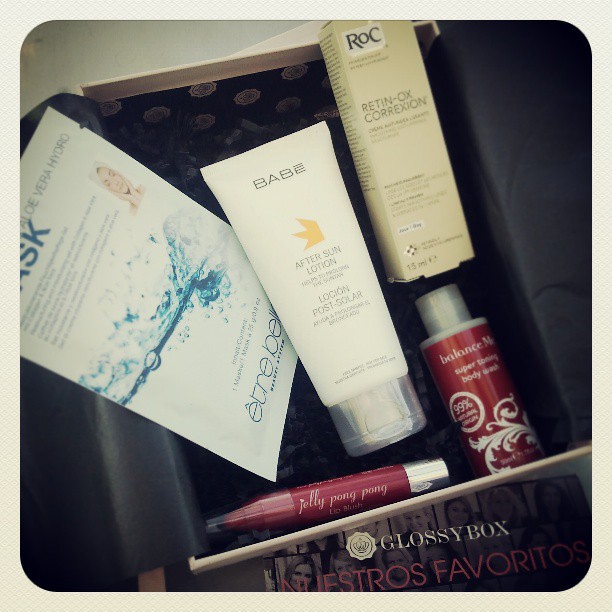The image depicts an open, organized black makeup bag or case with small brown floral designs, containing a variety of beauty and skincare items. On the left side, there is a flat container labeled "Vera Hydro Mask" featuring blue and white splashing water graphics. Adjacent to it, in the center, is a white tube labeled "Babe After Sun Lotion," accompanied by a yellow icon above the text. Another prominent item is a gold box on the right side that reads "ROC" in blue letters in the top left corner and "Retin-OX Correction" in black letters below. Nearby is a small red container with a white label that says "Balance Me Super Toning Body Wash, 99%." Towards the lower left, there is a lip product marked "Jelly Pong Pong Lip Blush" featuring a red label. The interior of the bag includes smooth black packing paper, which adds to the overall neat presentation of the cosmetic products. The exterior of the box is labeled "Glossy Box, Nuestros Favoritos," indicating a curated selection of favorite items.